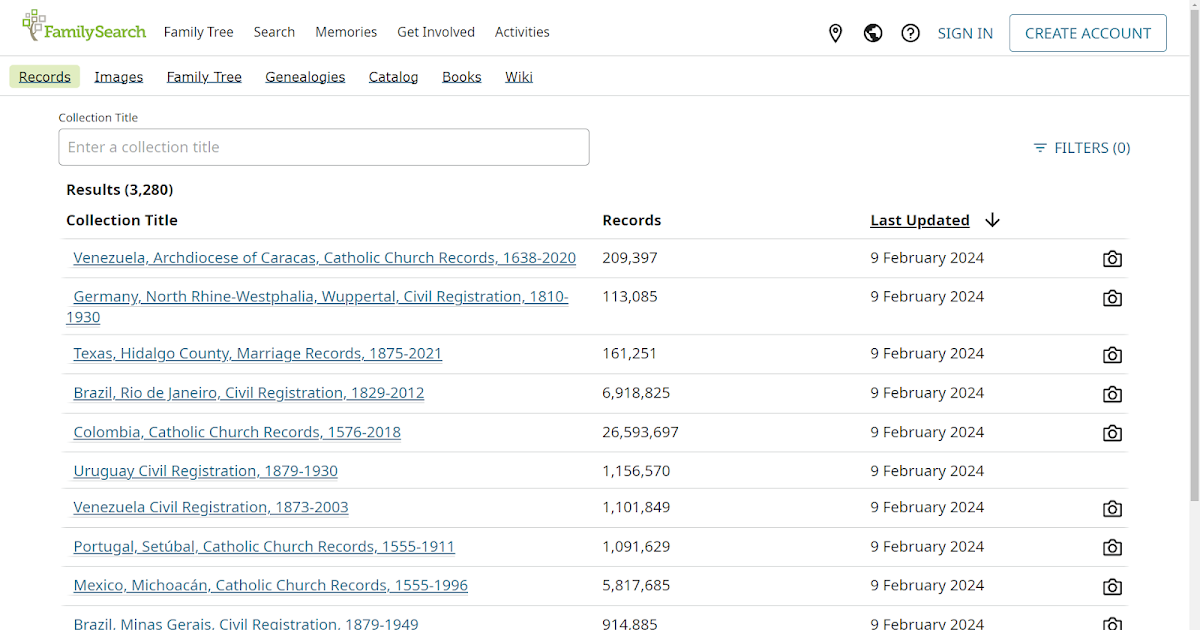The image depicts the homepage of FamilySearch, a genealogy website. In the upper left corner, there's an image of a tree next to the word "FamilySearch" in green. To the right, in small gray text, are the navigation options: FamilyTree, Search, Memories, Get Involved, and Activities. Further right, icons for location, a globe, and a help question mark appear, followed by "Sign In" in light blue text. Next to it is a white button outlined in gray that reads "Create Account."

Beneath this header, another navigation bar offers the options: Records, Images, FamilyTree, Genealogies, Catalog, Books, and Wiki. The "Records" option stands out with a green box around it.

Below this, a search field labeled "Collection Title" invites users to "Enter a Collection Title." The search results beneath this field show "Results: 3,280" in black text.

The results list displays at least ten records, each organized with the "Collection Title" on the left, followed by the number of records, and the date each was last updated.